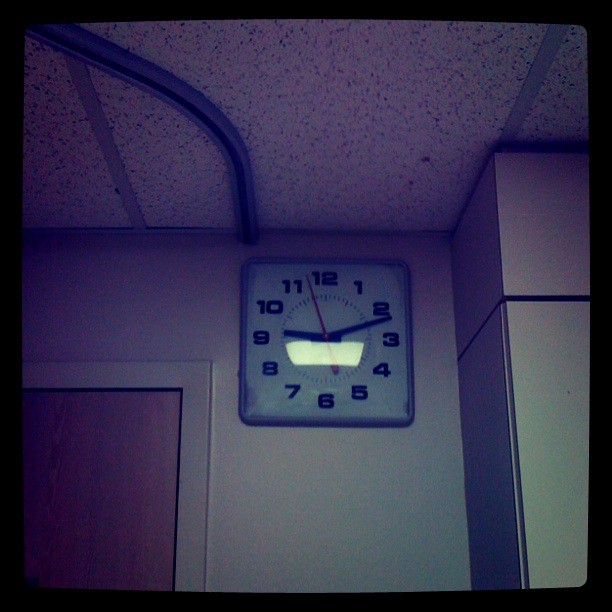The photo depicts a dimly-lit room with a slightly dated ambiance, characterized by drop ceilings made of foam-like panels set into metal strips. Dominating the scene is a square clock nestled high on the wall, almost touching the ceiling. The clock, which is unconventional in its square shape, features black hour and minute hands, along with black numbers from 1 to 12, while the second hand stands out in red. The time displayed is 9:12. To the right of the clock, a pillar is visible, contributing to the architectural depth of the space, which is bathed in a lilac-gray tint. To the left, there is a contrasting white door frame with a heavy light brown wooden door, adding to the vintage feel of the environment.